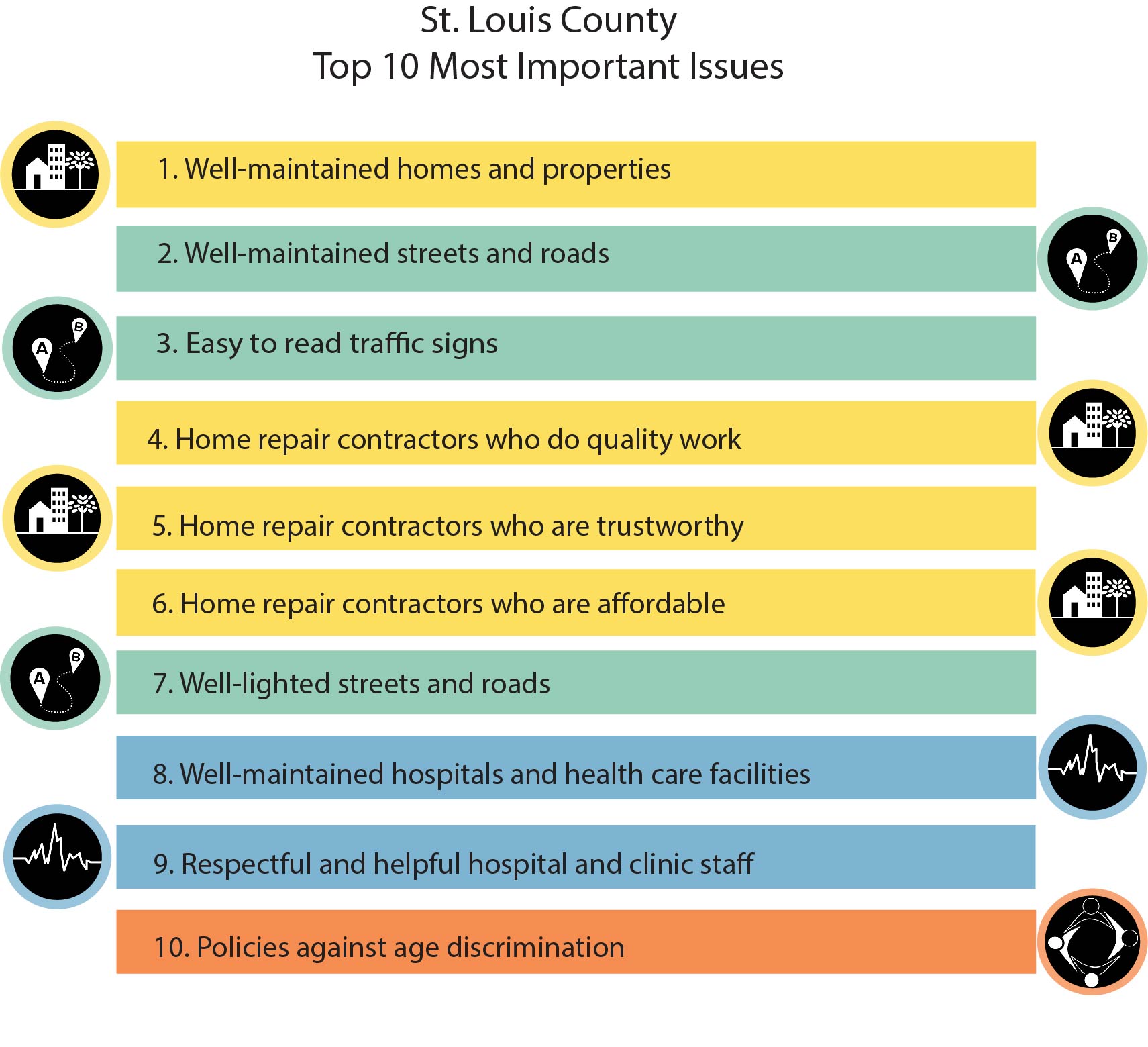In this infographic titled "St. Louis County: Top 10 Most Important Issues," a detailed visual layout showcases the key concerns in the area, using a color-coded system for clarity. The infographic features ten horizontal rectangles, each paired with a corresponding circular icon that has a black center with a white sketched design. These rectangles are numbered from 1 to 10 along the left side and alternate the position of their circles left and right. The colors used are yellow (for numbers 1, 4, 5, and 6), turquoise (for numbers 2, 3, and 7), aqua blue (for numbers 8 and 9), and orange (for number 10).

1. **Well-Maintained Homes and Properties** - Yellow, with a circle on the left showing a house, apartment building, and tree.
2. **Well-Maintained Streets and Roads** - Turquoise, circle on the right showing points A to B with a path.
3. **Easy to Read Traffic Signs** - Turquoise, circle on the left with the same A to B symbol.
4. **Home Repair Contractors Who Do Quality Work** - Yellow, circle on the right depicting a house, apartment, and tree.
5. **Home Repair Contractors Who Are Trustworthy** - Yellow, circle on the left with a similar design of house and tree.
6. **Home Repair Contractors Who Are Affordable** - Yellow, circle on the right with the familiar house and tree.
7. **Well-Light Streets and Roads** - Turquoise, circle on the left with the A to B symbol.
8. **Well-Maintained Hospitals and Healthcare Facilities** - Aqua blue, circle on the right featuring an EKG lifeline.
9. **Respectful and Helpful Hospital and Clinic Staff** - Aqua blue, circle on the left also showing the EKG design.
10. **Policies Against Age Discrimination** - Orange, circle on the right illustrating heads and arms linked in a circle, alternating in black and white.

Each rectangle clearly labels one of the top 10 issues identified as priorities, with the alternating circular icons adding visual cues to represent each issue.